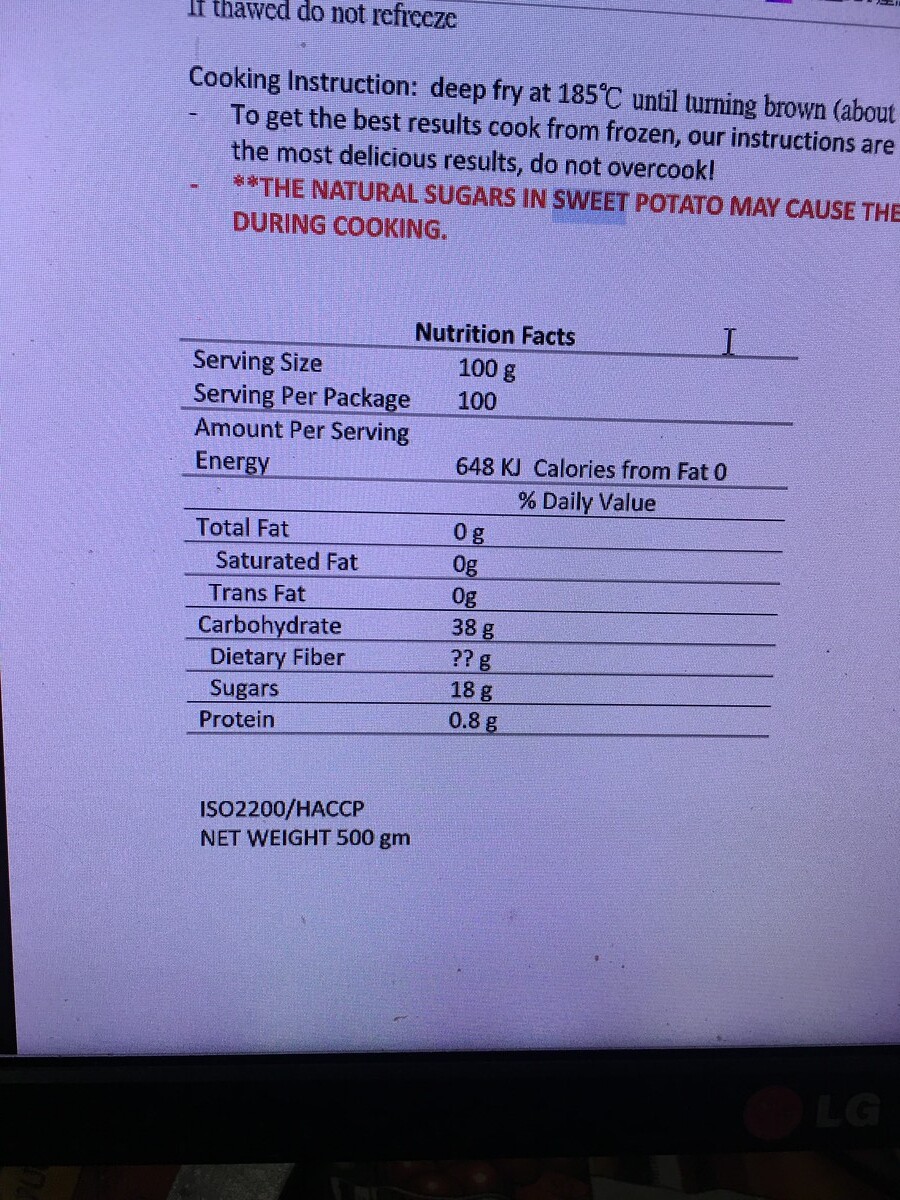The image depicts a white piece of paper containing detailed cooking instructions and nutritional information for sweet potato fries. From top to bottom, the text reads:

- "If thawed do not freeze."
- "Cooking Instructions: Deep fry at 185 degrees Celsius until turning brown. For best results, cook from frozen. Do not overcook." This part is highlighted in red.

Below the instructions, the nutrition facts for sweet potatoes are provided:

- Serving size: 100 grams
- Servings per package: 1
- Total fat: 0 grams (includes no saturated fat and no trans fat)
- Carbohydrates: 38 grams
- Dietary fiber: [Information appears to be incomplete or marked by a question mark]
- Sugars: 18 grams

There is a mention of natural sugars in sweet potatoes causing something during cooking, but the text is cut off and incomplete.